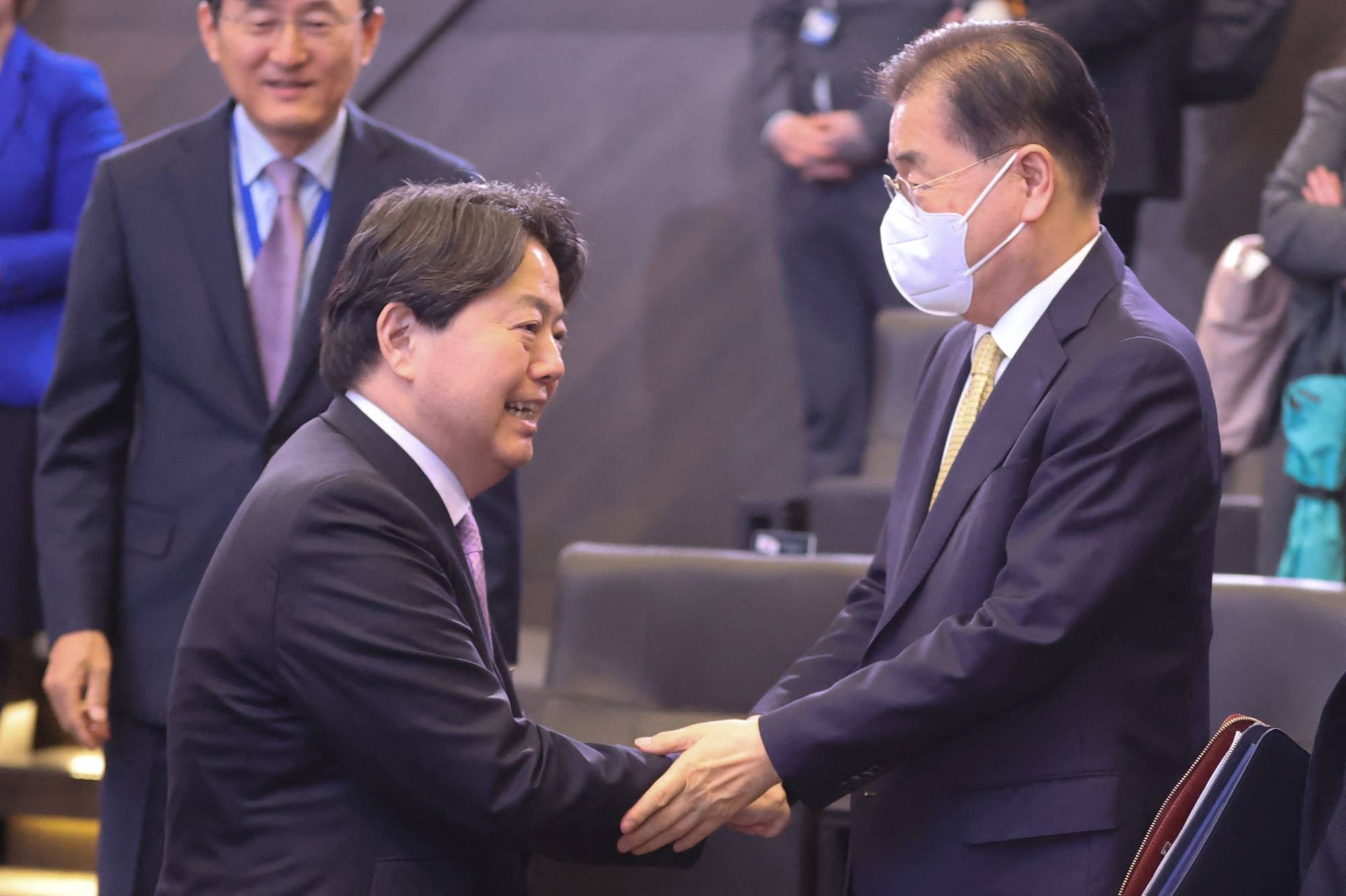In this photograph, two East Asian gentlemen, possibly Chinese or Korean politicians, are the main subjects, captured mid-handshake. Both are dressed in dark suits. The man on the left, slightly turned to his right, sports a pink tie and white shirt, and has a slight smile on his face. His right arm is extended to shake hands with the man on the right, who faces left, and wears a white face mask, glasses, a white shirt, and a yellow tie. His left hand rests on the arm of the man he is shaking hands with. They seem to be engaged in a formal yet somewhat casual meeting, likely at a conference or political event. In the background, a brown wall and several slightly blurred figures from the waist down can be seen, along with another man standing with small glasses, hands at his sides, observing the interaction. The background also includes gray or black chairs, adding to the conference-like atmosphere.